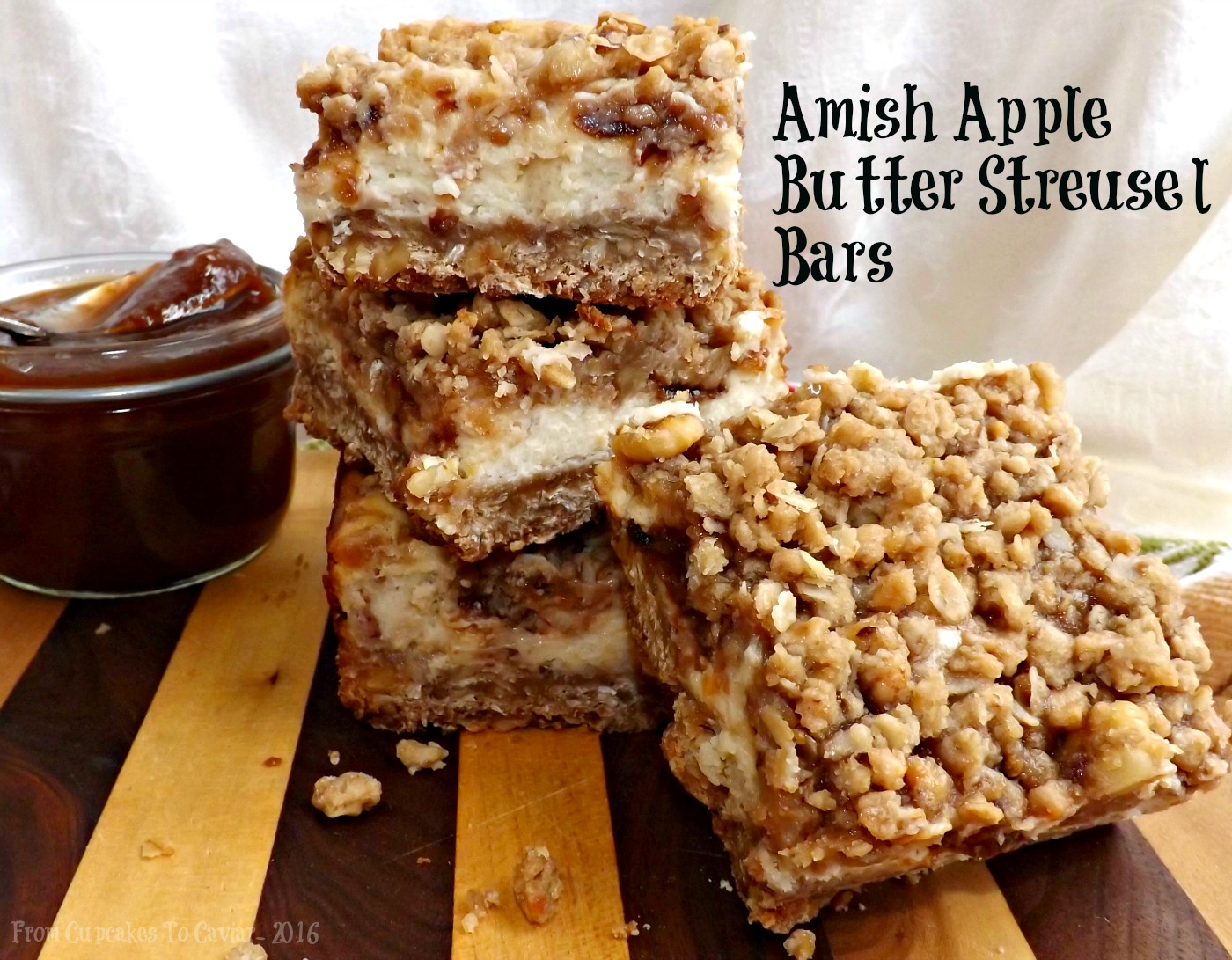The image showcases a delectable display of Amish Apple Butter Streusel Bars meticulously cut into squares, with a central stack of three bars and a fourth bar positioned in front of the stack. The bars feature a layered composition: a darker bottom, a lighter middle, and a topping that appears to include nuts or a crunchy granola-like texture. The scene is set on a striped surface of brown and yellow hues, possibly a cutting board or countertop. To the left, there is a glass bowl containing a brown, jelly-like apple butter with a spoon resting inside. The background is adorned with a white cloth. Text appears at two corners of the image: "Amish Apple Butter Streusel Bars" is written in black at the top right, and "From Cupcakes to Caviar 2016" is inscribed in white at the bottom left.